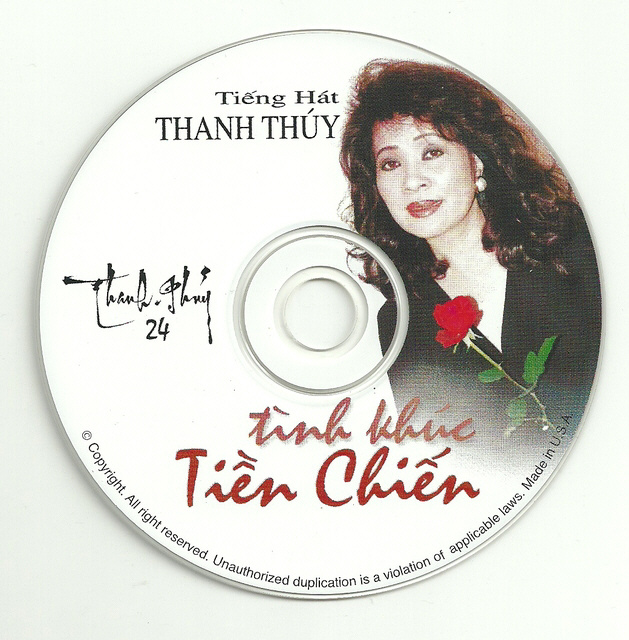The image shows a CD set against a white background. On the right side of the CD, there is a photograph of a woman with long, dark hair and Asian features. She is holding a red rose in front of her chest and wearing a black V-neck dress, complemented by red lipstick. To the upper left of the woman’s head, the text "Tieng Hat Thanh Thuy" is displayed. Just to the left of the CD's center hole, there is a black script signature "Thanh Thuy" followed by the number "24." Below the inner ring of the CD, the name "Thien Kieu" can be seen, and across the bottom in red script font, the name is repeated with the phrase "Tieng Chien." Additionally, at the bottom edge of the CD, there is a semi-circular footnote indicating copyright information, stating "All rights reserved," and notes on unauthorized duplication being a violation of applicable laws, made in the USA. The overall design is a detailed photographic representation emphasizing realism and package design.